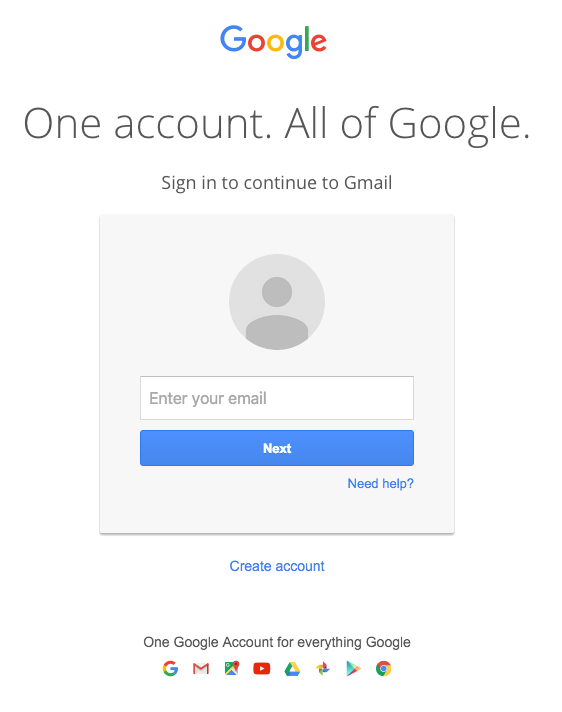The image is a screenshot from a device, either a phone or a computer, showcasing the Google sign-in page. Prominently displayed in the upper center are the colorful Google letters. Below this, in gray text, it reads, "One account. All of Google." Underneath, in smaller text, is the instruction, "Sign in to continue to Gmail."

Central to the image is a light gray square. At the top of this square, there is a gray circle containing a simplistic icon of a person's head and body. Beneath this, there is a white input box with the prompt, "Enter your email." Below the input box is a blue bar labeled "Next," which user can click to proceed.

In the bottom right corner of the gray square, the text "Need help?" follows a question mark. Just outside the gray square and beneath it, the phrase "Create account" appears in blue, indicating a clickable link to set up a new account. 

At the very bottom of the image, the statement "One Google account for everything Google" is written in black text. Beneath this sentence is a row of various Google product symbols, including the recognizable "G" for Gmail, a red "M", a red rectangle with a white play button for YouTube, and the Google Chrome emblem, among others.